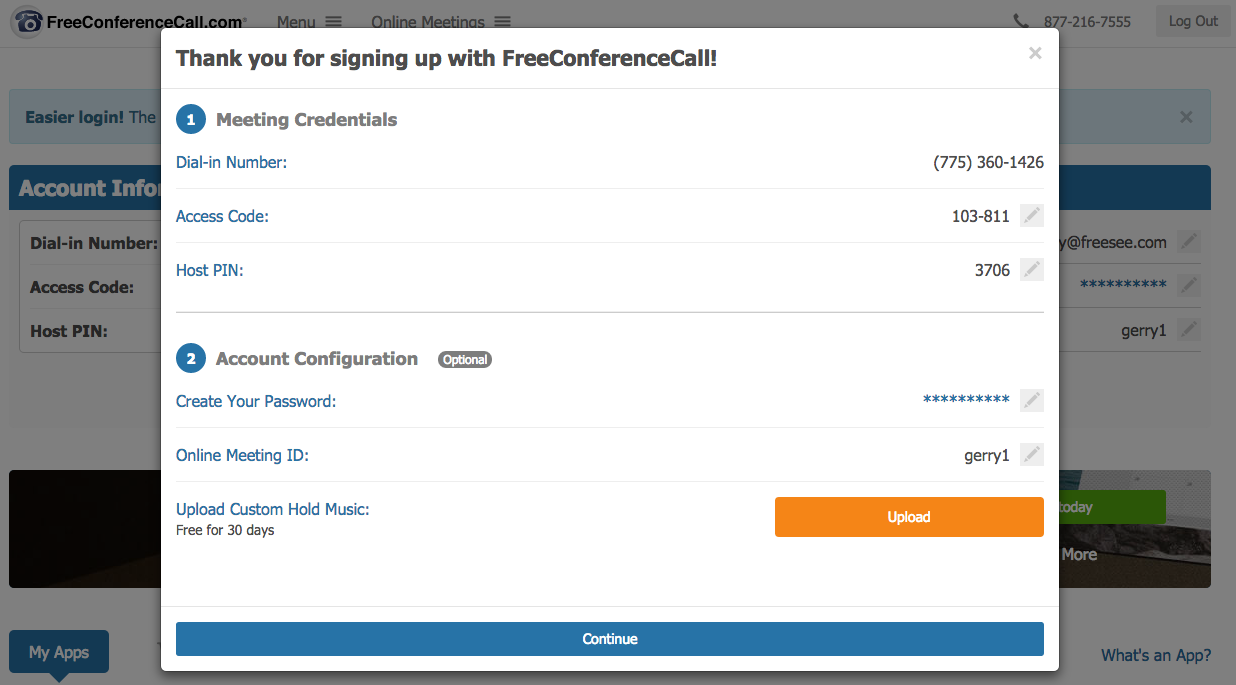The image is a screenshot of the Free Conference Call website, with the main content partially obscured by a darkened overlay. At the top of the blurred background, the website's header is visible, displaying the FreeConferenceCall.com logo along with menu options such as "Online Meetings" on the left and a phone icon with the number 877-216-7555 on the right. Additionally, there is a "Log Up" option located here.

Dominating the center of the screen is a pop-up notification box with a black header containing the message "Thank you for signing up with Free Conference Call!" with the "Free Conference Call" text formatted as a single word with capital letters F, C, and C.

Below this header, a blue circular icon with a white number "1" inside introduces the section titled "Meeting Credentials" in gray text. The section provides a dial-in number (775-360-1426), an access code (103-811), and a host pin (3706).

Further down, a blue circular icon with the number "2" in white signifies the "Account Configuration" section, labeled as "optional" in a gray banner with white text. This section allows users to create a password, set up an online meeting ID, and upload custom hold music, which is offered free for 30 days. Below this, an orange button with white text reads "Upload."

At the very bottom of the pop-up is a blue background strip featuring a white "Continue" button for users to proceed further.